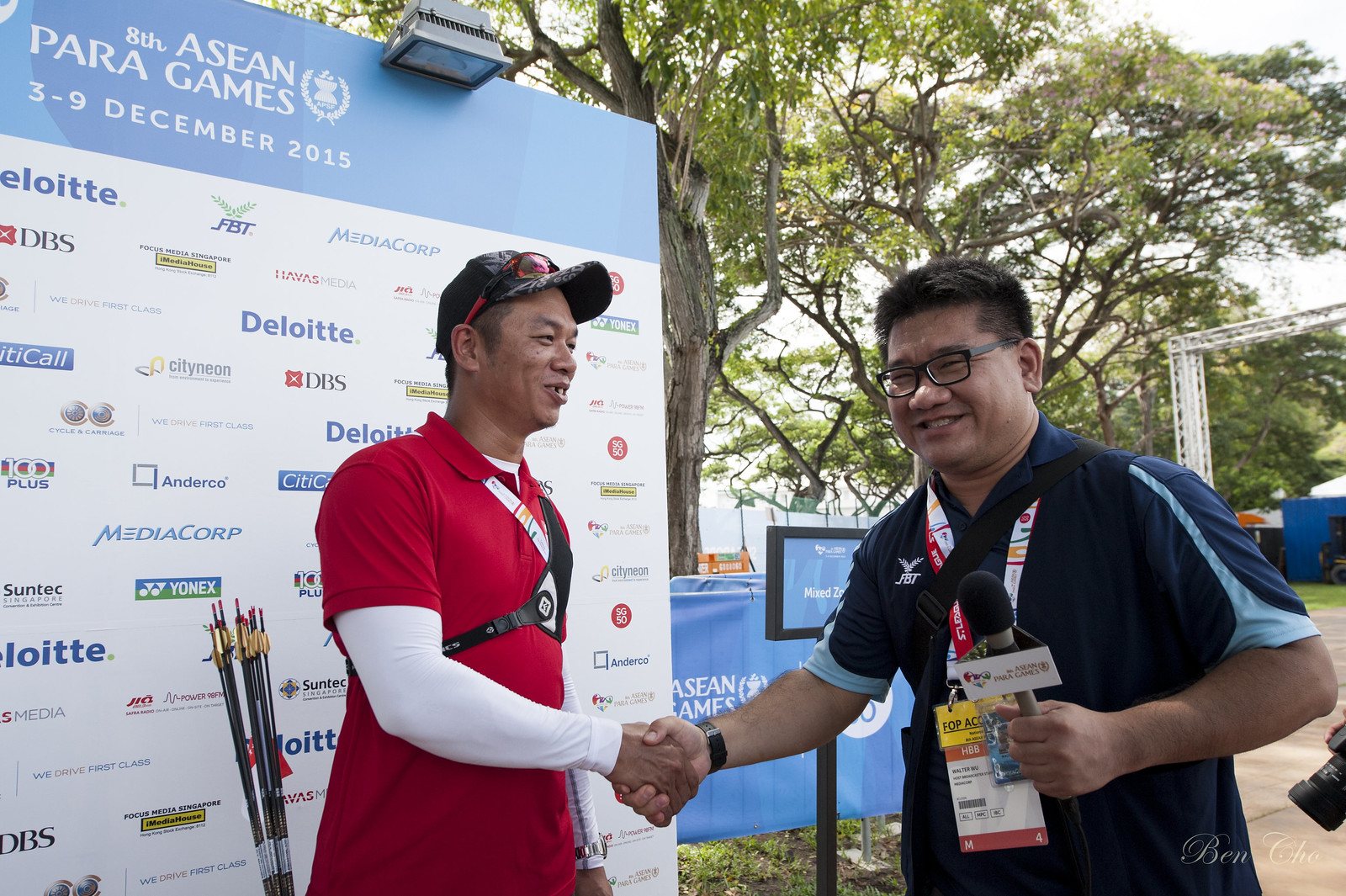This outdoor photograph captures a moment of camaraderie between two men shaking hands. The man on the right, smiling and facing the camera, wears glasses and has short brown hair. He's dressed in a dark blue and light blue JBT shirt and holds a microphone emblazoned with "ACN Paragames" in gold text. Around his neck hang several badges, prominently displaying an "FOP access" badge. The man on the left, who is facing the other man, appears to be in his 40s. He sports a black baseball cap with red and black sunglasses perched on top, a red polo shirt over a white long-sleeved undershirt, and some type of black shoulder gear. Behind him on the ground are arrows. The background features a white board displaying numerous corporate logos, with a banner at the top reading "8th ACN Paragames, 3-9 December 2015." The setting is outdoors, evident from the visible trees behind them.